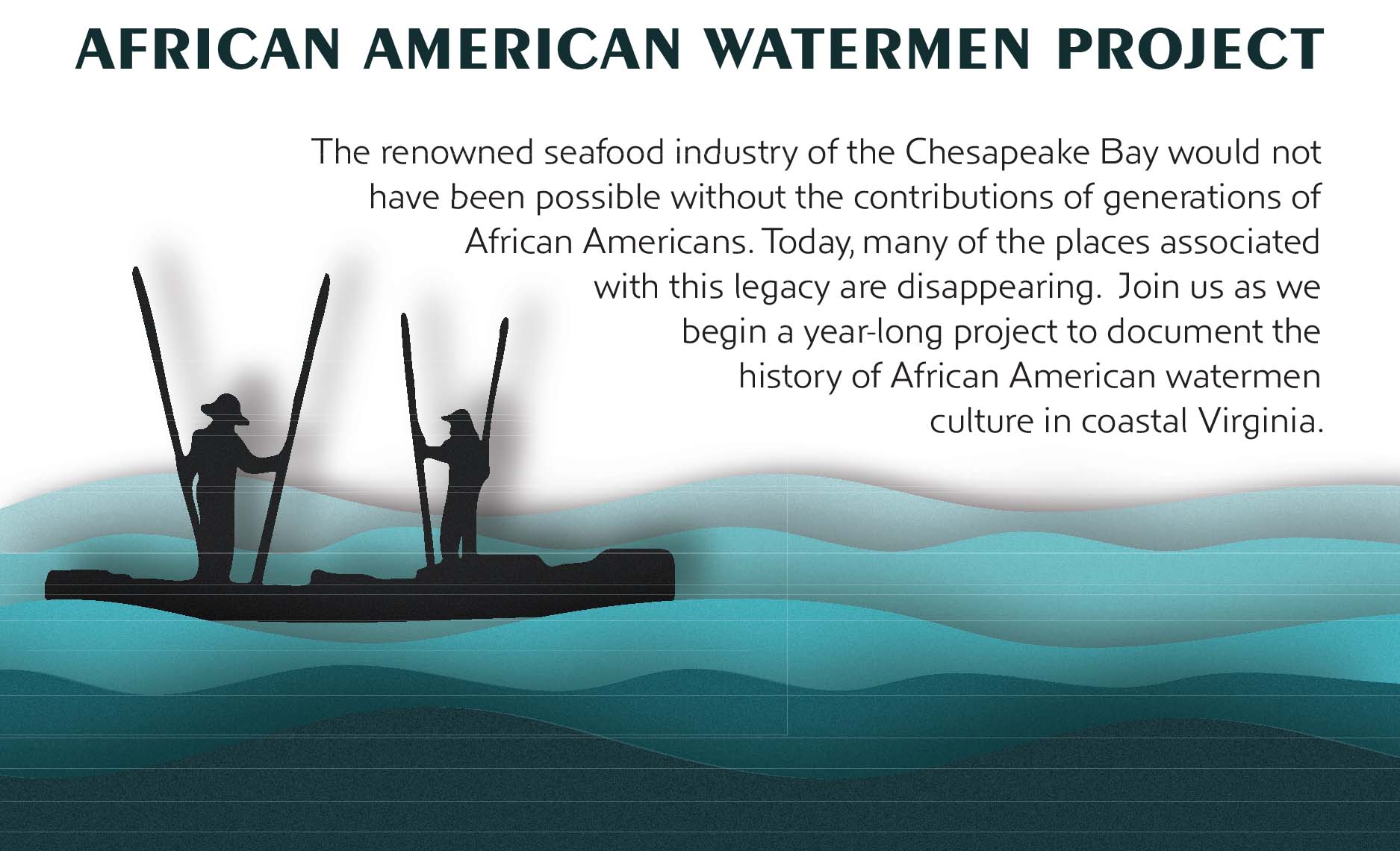The poster titled "African American Watermen Project" features a prominent black text header, set against a white background. Under the headline, it reads, "The renowned seafood industry of the Chesapeake Bay would not have been possible without the contributions of generations of African Americans. Today, many of the places associated with this legacy are disappearing. Join us as we begin a year-long project to document the history of African American watermen culture in coastal Virginia." At the bottom part of the poster is an artistic image of water, transitioning from light blue teal at the top to a darker blue at the bottom. On the left side, silhouetted in black, are two figures standing on boats. One figure wears a baseball cap, and the other a fisherman hat, and both hold long poles. The scene is further defined by multiple shades of green waves. The figures, indistinguishable in gender and devoid of facial details, contribute to the historical and cultural narrative depicted in this evocative poster.